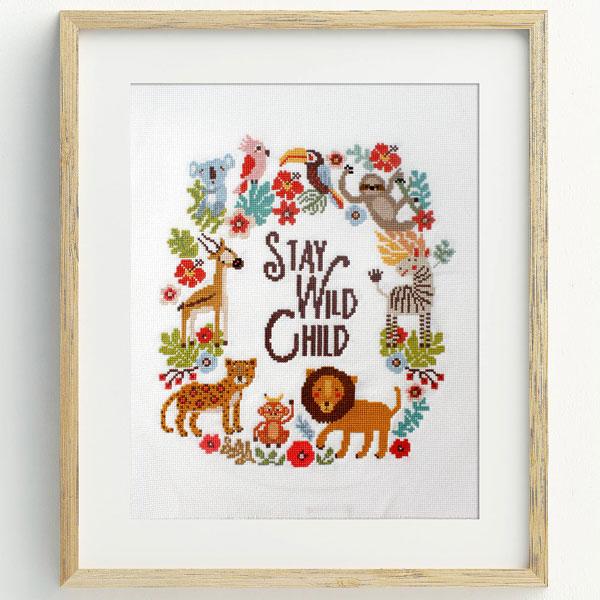This image is a square, four-inch by four-inch piece of framed cross-stitch artwork. Encased in a light brown wooden frame with a white matting border, the design sets against a plain white background. At the very center of the cross-stitch, in dark brown text, are the words "Stay Wild Child." Encircling this central text are various colorful animals: starting at the top is a toucan, followed by a sloth to its right. Further clockwise at the three o'clock position is a zebra, below which, at six o'clock, resides a lion. Moving leftwards, we encounter a monkey adorned with a small crown, succeeded by a cheetah. Positioned at nine o'clock is an antelope, above which is a koala and a pink parrot. These animals are interspersed with vibrant decor elements including red, pink, and blue flowers, along with various green and teal leaves, creating a visually appealing yet minimalistic composition.